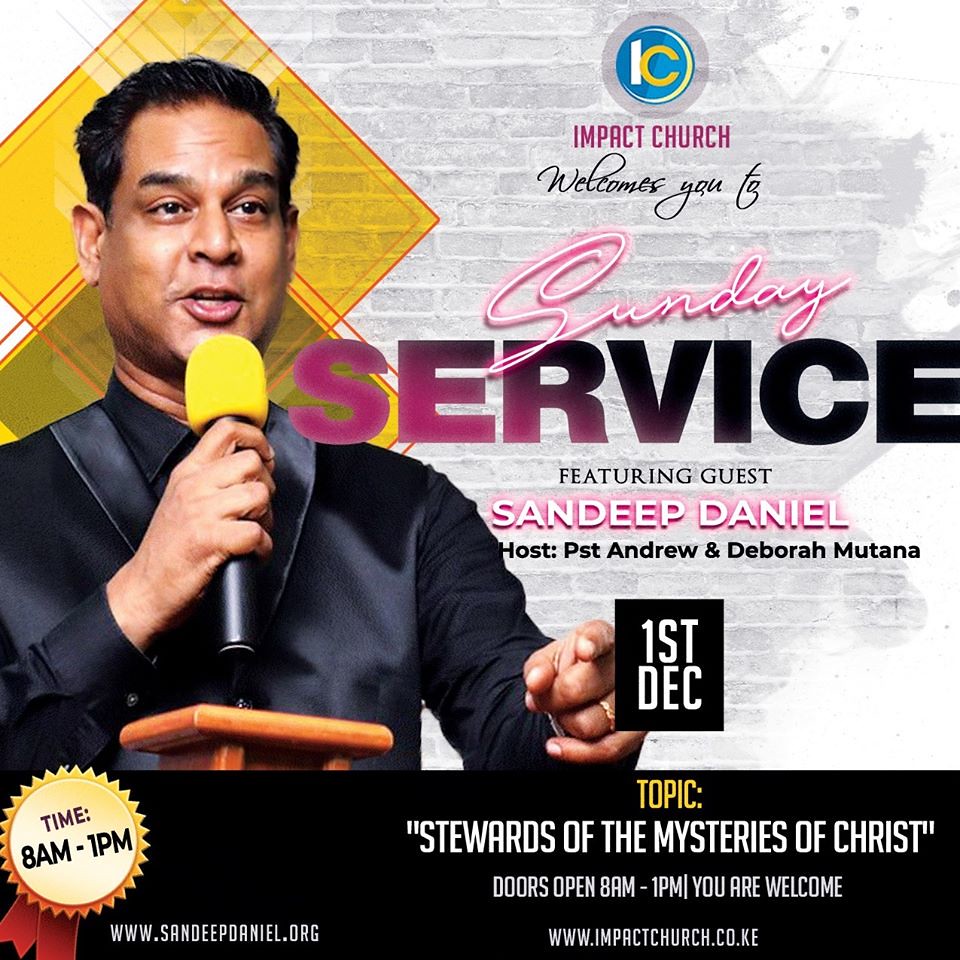The promotional flyer from Impact Church prominently features an event announcement for their Sunday service on December 1st. The left side of the image depicts an Indian man in a sleek, black silk suit with shiny lapels, a yellow hat, and a matching microphone with a yellow mouthpiece. He is speaking and pointing forward with his left hand. His name is Sandeep Daniel, the guest speaker for the service. The flyer text, written in neon cursive and black and mauve gradients, reads: "Impact Church welcomes you to Sunday service featuring guest Sandeep Daniel, hosted by Pastor Andrew and Deborah Mutana." The service is scheduled from 8 a.m. to 1 p.m., with the topic titled "Stewards of the Mysteries of Christ." The flyer provides additional details with the websites www.impactchurch.co.ke and www.sandeepdaniel.org, inviting everyone to join the service.